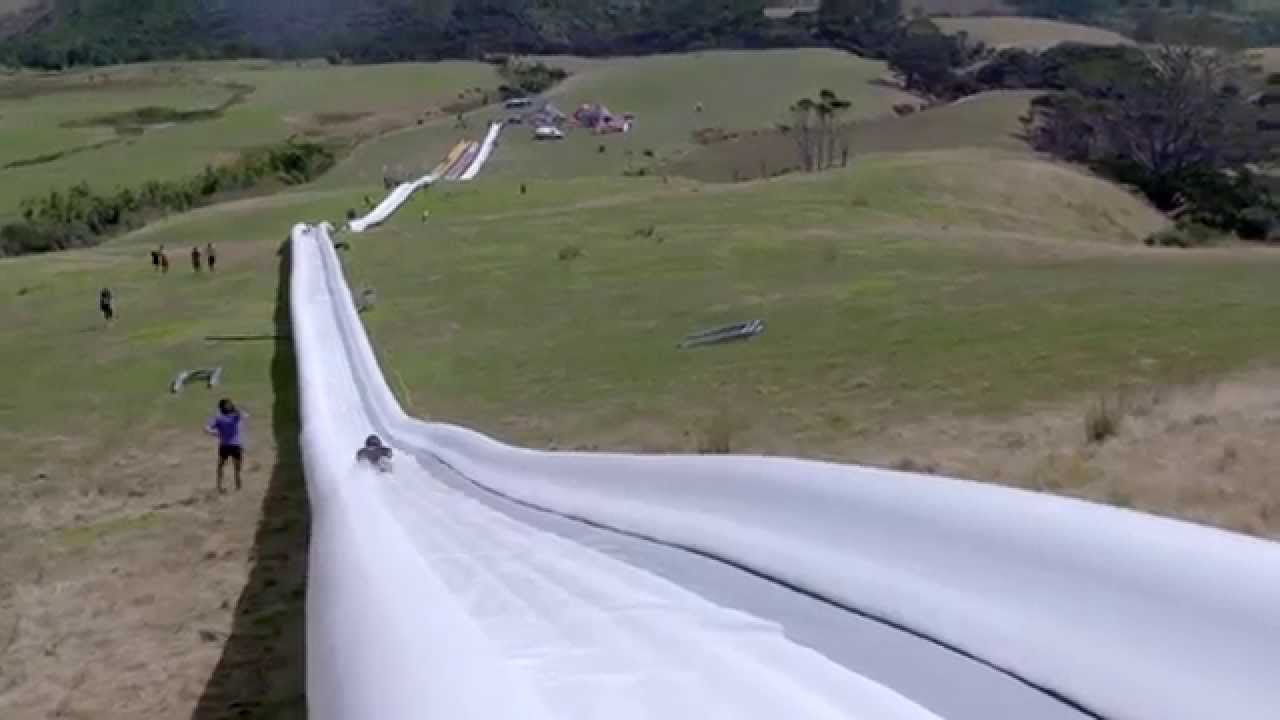A sprawling, white water slide stretches down a grassy hill, potentially holding the world record for the longest slide ever. The perspective from the top allows a sweeping view over a landscape rich with dense, dark green trees, with occasional patches of brown in the grass. The slide weaves its way far into the distance, where a festival seems to be taking place at the bottom of the hill. A person, belly down, is in the midst of their thrilling descent, while several others either walk uphill or downhill alongside the slide. The bright daylight enhances the vibrancy of the scene, capturing an adventurous moment overseen by a supervisor near the top left of the image.